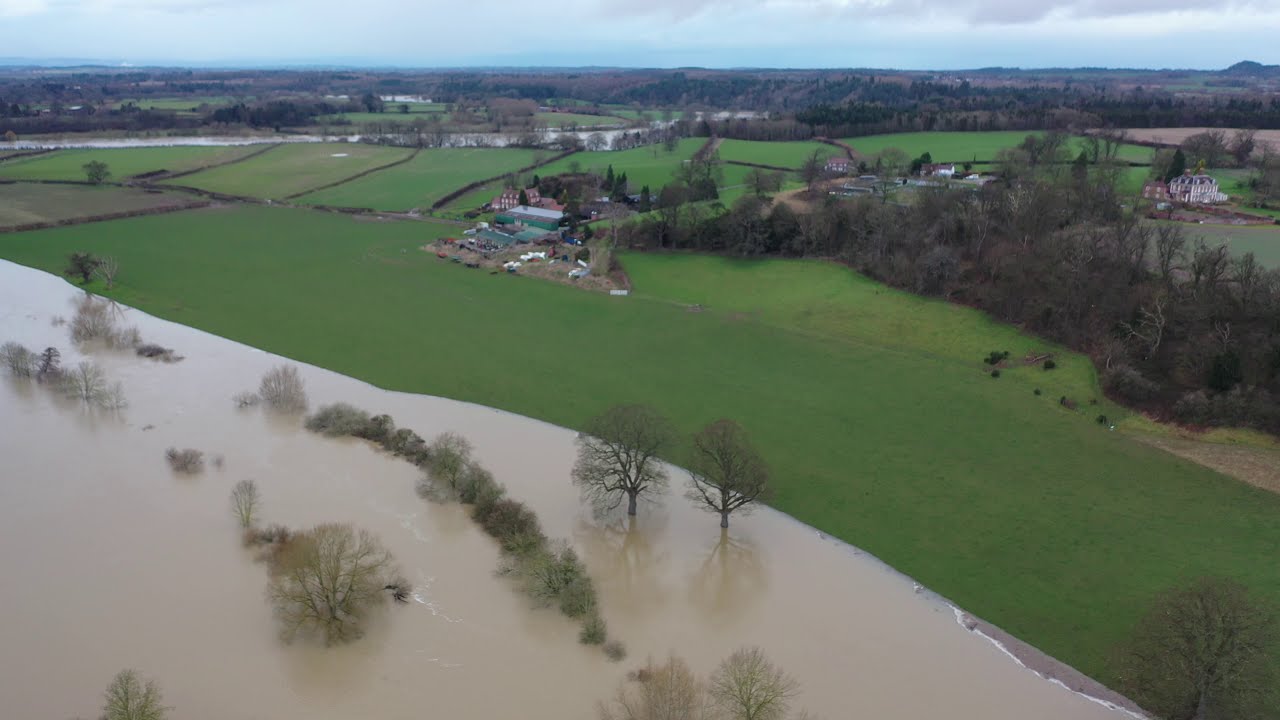The photograph captures a panoramic view of a rural landscape, revealing a recent flood. From the bottom right to the middle left of the image, a large, muddy expanse of water inundates the land, submerging trees and bushes. Adjacent to this floodwater, a green pasture stretches to the right, with distant buildings, likely houses, dotting the scene. Further right and extending upwards, a dense tree line separates this area from more segmented green plots and additional structures. The upper part of the image showcases divided parcels of lush grassland with brown borders, giving way to a winding river that flows right to left across the top, hinting at its contribution to the flooding below. In the distant horizon, faint silhouettes of trees, grasslands, and buildings emerge under a cloudy, overcast sky, with hills and more trees occupying the upper right portion, completing this detailed and serene yet impacted rural tableau.